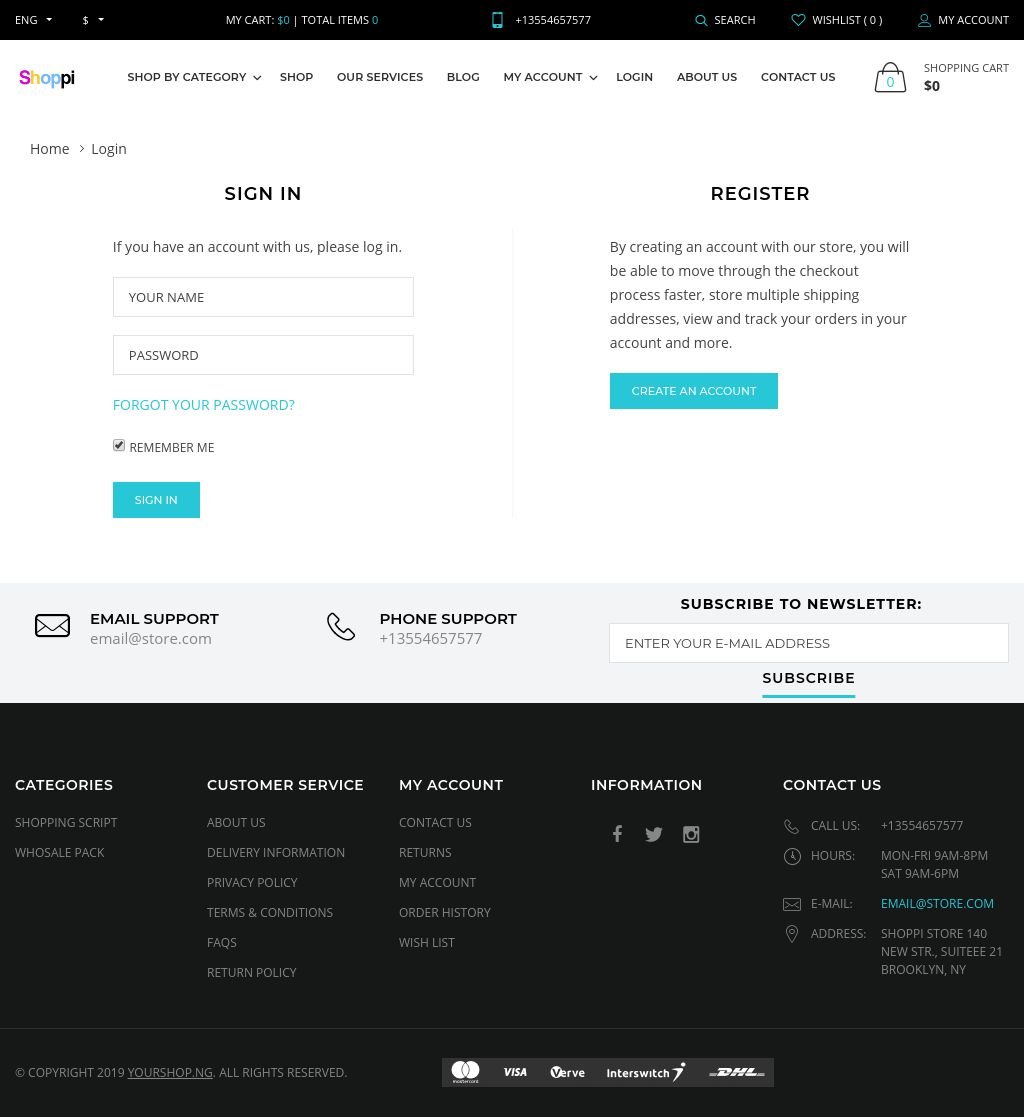This image appears to be a screenshot of an e-commerce website displayed on a laptop or desktop computer, formatted as a slightly taller-than-wide rectangle. The top of the image features a black navigation bar with slightly bunched-up text, including a drop-down menu icon and a segment that reads "My Cart" followed by a green "0," indicating an empty shopping cart. Beside it, a green "0" also notes zero total items.

Prominently in the center, a green cell phone icon accompanied by white text displays a support phone number. To the left, the site’s logo, "Shopei" (spelled S-H-O-P-E-I), is colorfully presented in pink, yellow, blue, and black lettering.

Directly beneath the logo, there are several navigation options that seem to be "Shop by Category" and "Shop," though some of the text is unreadable due to font compression. The next section contains a menu with links likely titled "Home" and "Login."

Below this menu, the website features a sign-in form header, prompting users to enter their name and password. This section includes a blue "Sign In" button at the bottom and a pre-checked "Remember Me" box. Adjacent to this, there's an option for new users to register, highlighted by a "Register" button and a blue box with the phrase "Create Account" in white font.

At the very bottom of the screen, there are icons for email support, phone support, and a subscription to the newsletter, suggesting multiple options for user assistance and engagement.